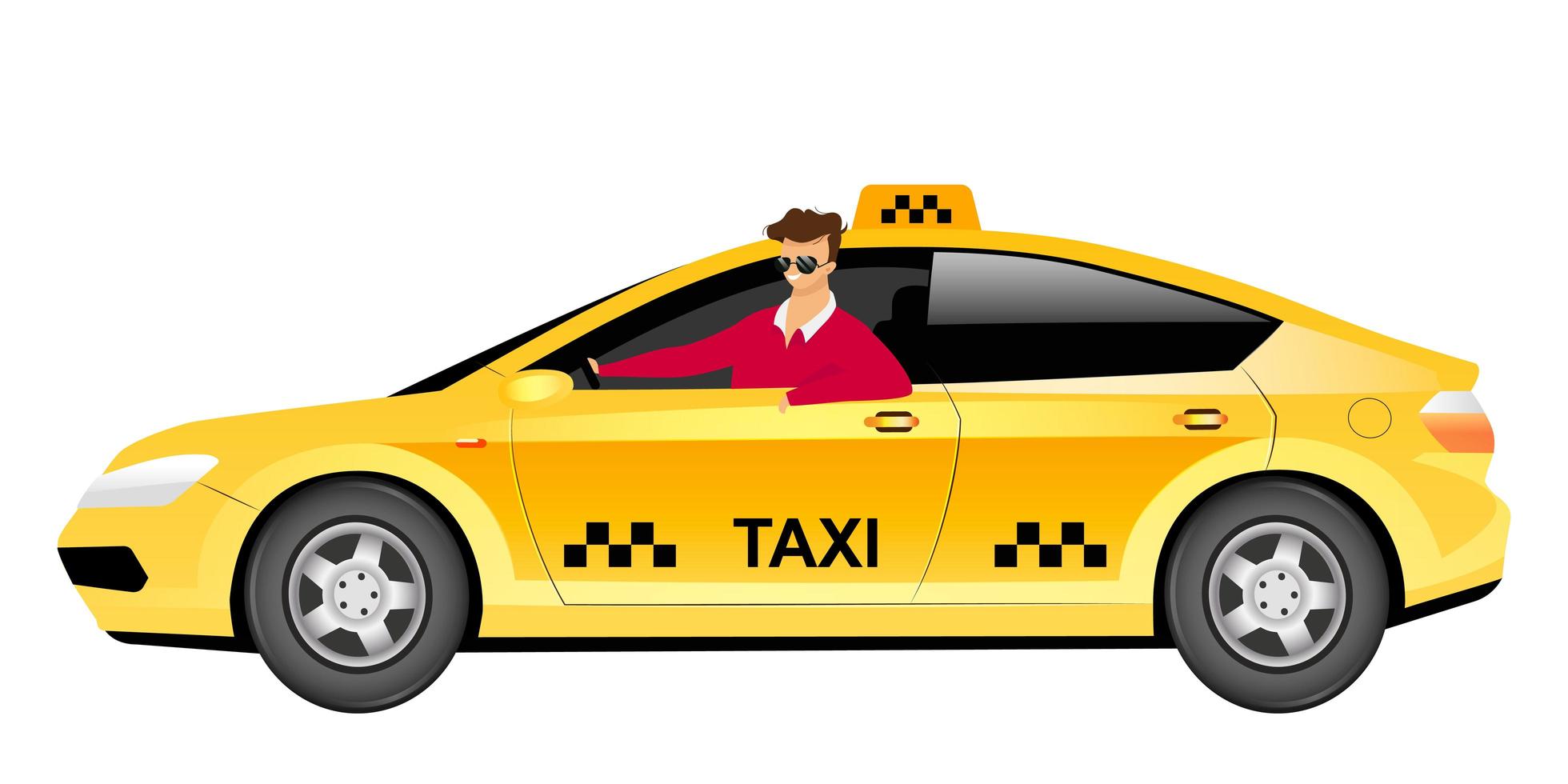In the illustration, a bright yellow, modern four-door sedan taxi is depicted against a white background. The taxi is immaculately clean and features vibrant colors. The word "TAXI" is prominently displayed on both the driver's door and a signage board atop the vehicle, which is also adorned with a distinctive checkerboard pattern. The car has silver wheels, tinted black windows, and visible headlights, taillights, and a gas cap.

The driver, a man with short brown wavy hair and black glasses, is leaning out of the driver's side window. He appears to be Caucasian and is wearing a red sweater over a white collared shirt. His left arm is resting on the door, and his right arm is positioned on the steering wheel, while his head extends entirely outside the window.